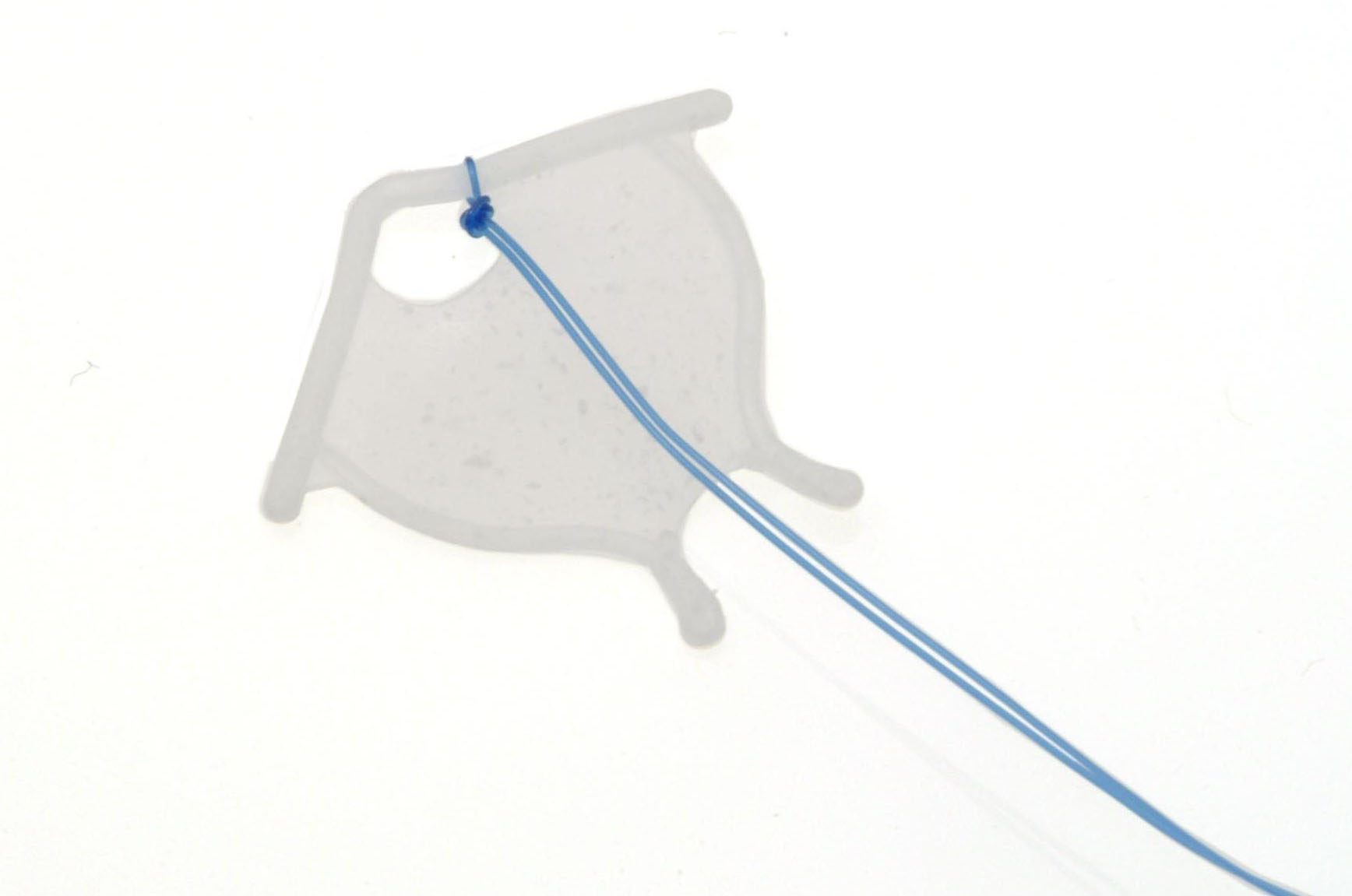The image showcases a white, kite-shaped medical device that resembles a stingray or a butterfly with a unique, asymmetrical form. The device appears to be made of plastic or silicone and has a pitched, roof-like top. At the top center, there is a circular opening through which a blue wire is threaded, creating a knot. This blue wire splits into two strands extending off to the bottom right of the image. The entire device is placed against a white background, with the wire casting a shadow below. The object also features darker white specks all over its surface, which do not obscure the more prominently outlined white edges. The photo, taken with overhead lighting, captures the detailed contours and the intricate construction of the device.